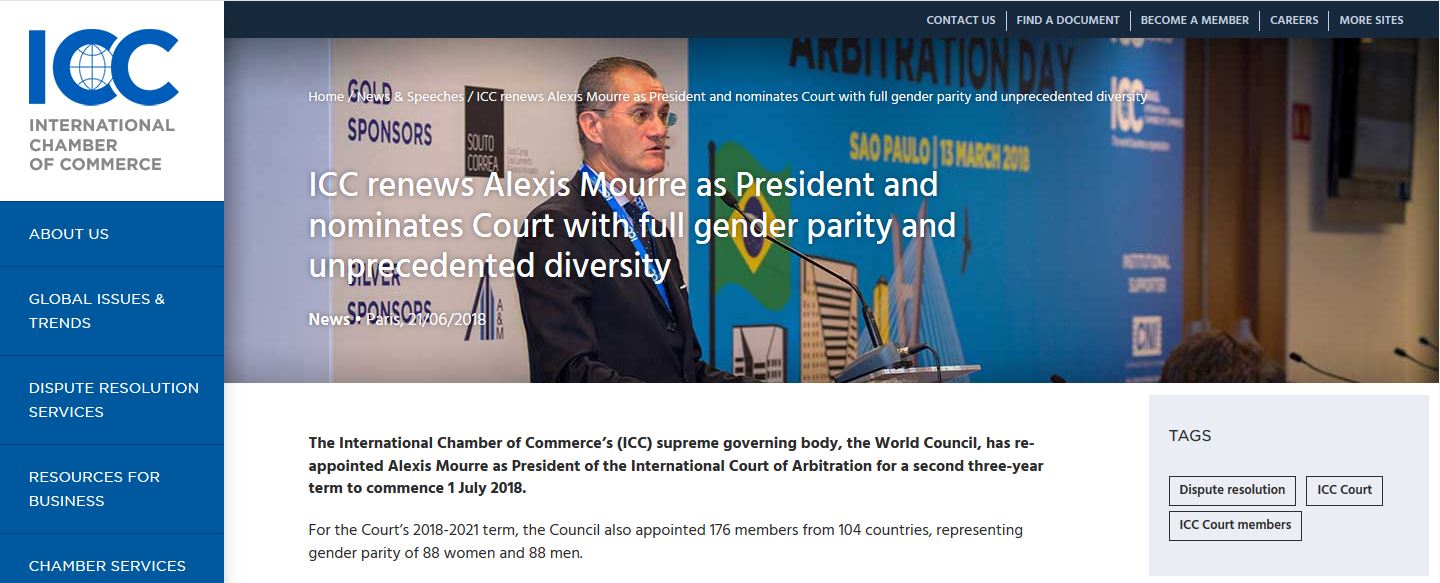In this detailed image, the left-hand side showcases a white box with prominent blue lettering that reads "IOC," featuring a world map in blue within the "O." Below this, it says "International Chamber of Commerce" in gray letters. Adjacent is a large blue box divided into three sections: the first section, in light blue print, reads "About Us Global Issues and Trends"; the second section details "Dispute Resolution Services"; and the third section mentions "Resources for Businesses" and "Chamber Services."

On the right-hand side of the image, there's a photograph of a man in a dark suit with a blue tie, wearing glasses, standing against a white wall that displays "Gold Sponsors" along with some numbers. Next to this is a blue wall with the text "Arbitration Day" in black, accompanied by the number "100" in white. Below this, "Sao Paulo, March 2018" is written in yellow, and additional white text. A white box at the bottom contains "CN" in blue.

Further elements in the image include a green flag with yellow and black colors, a computer, and various other objects. Prominently displayed in white text is the headline "ICC Renews Alexis Moore as President and Nominates Court with Full Gender Parity and Unprecedented Diversity," followed by "News Paris 2006 to 2018." An article states, "The International Chamber of Commerce's supreme governing body, the World Council, has reappointed Alexis Murray as President of the International Court of Arbitration for a second three-year term to commence July 1, 2018."

Lastly, a small blue box labeled "Tags" contains three black boxes with the tags "Dispute Resolution," "ICC Court," and "ICC Court Members."